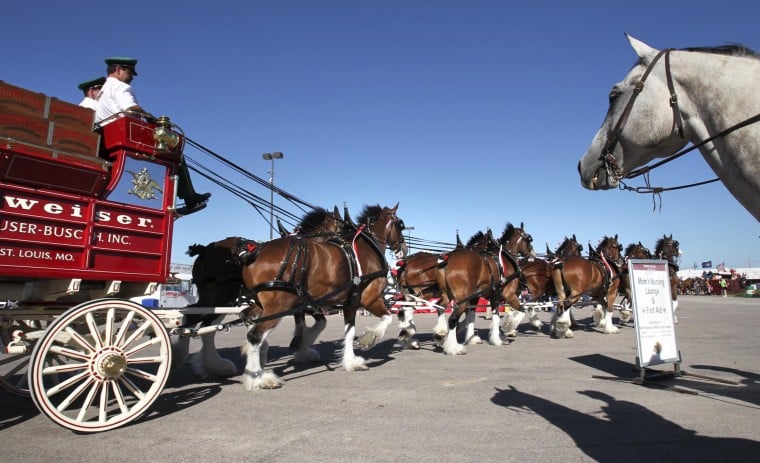In this detailed daytime photograph, a striking team of ten majestic Clydesdale horses is pulling a vibrant red Budweiser wagon, emblazoned with the words "Budweiser" and "Anheuser-Busch Inc., St. Louis, Missouri" in white text. The wagon features distinct white wheels and is being driven by two men dressed in white shirts, black pants, and brimmed hats. The clear, blue sky offers a perfect backdrop for the scene, suggesting a sunny afternoon with no clouds in sight. The image captures the horses in mid-motion, showcasing their strength and grandeur as they walk on a cement surface. Additionally, a separate white horse's head and neck are visible on the left side of the image, hinting at its presence at the event, though it's not part of the main team. This photograph likely depicts a parade or special event celebrating the iconic Budweiser Clydesdales.